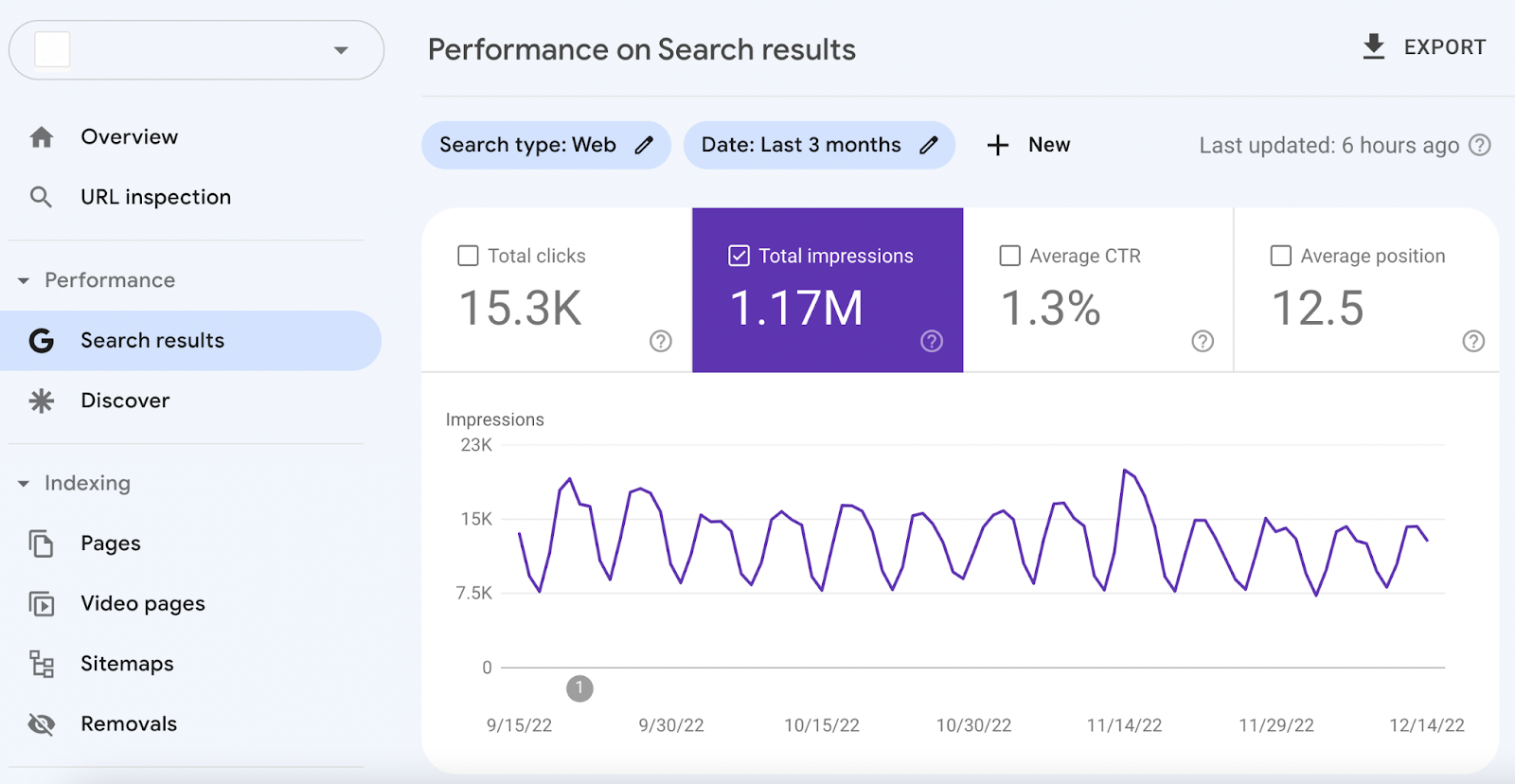**Detailed Caption:**

The image showcases a screenshot of a website performance interface with a pale blue background. At the top, a drop-down menu contains a small white square. To the left of the menu, a sidebar features various navigation options, starting with a house icon labeled "Overview," followed by a magnifying glass icon labeled "URL inspection." Below these are expandable sections for "Performance," "Search Results," and "Discover." The "Indexing" section, indicated by a downward arrow, lists subsections including "Pages," "Video Pages," "Sitemaps," and "Removals."

Centered at the top of the main panel is the title "Performance on Search Results," accompanied by a downward arrow and an "EXPORT" button in all capital letters. Beneath this, the interface displays filters within a long oval shape, labeled "Search Type: Web" and "Date: Last 3 Months," each with a pencil icon for editing. Adjacent to these is a "+ New" button.

A status note reads "Last updated 6 months ago." Below, a white panel summarizes key metrics: "Total Clicks: 15.3K," "Total Impressions: 1.17M" (highlighted against a purple background), "Average CTR: 1.3%," and "Average Position: 12.5."

Finally, a graph depicting changes in impressions over time spans the bottom of the panel. The vertical axis is marked with values (23K, 15K, 7.5K), and along the horizontal axis are dates: "09/05/2022, 09/15/2022, 09/30/2022, 10/15/2022, 10/30/2022, 11/14/2022, 11/29/2022, and 12/14/2022."